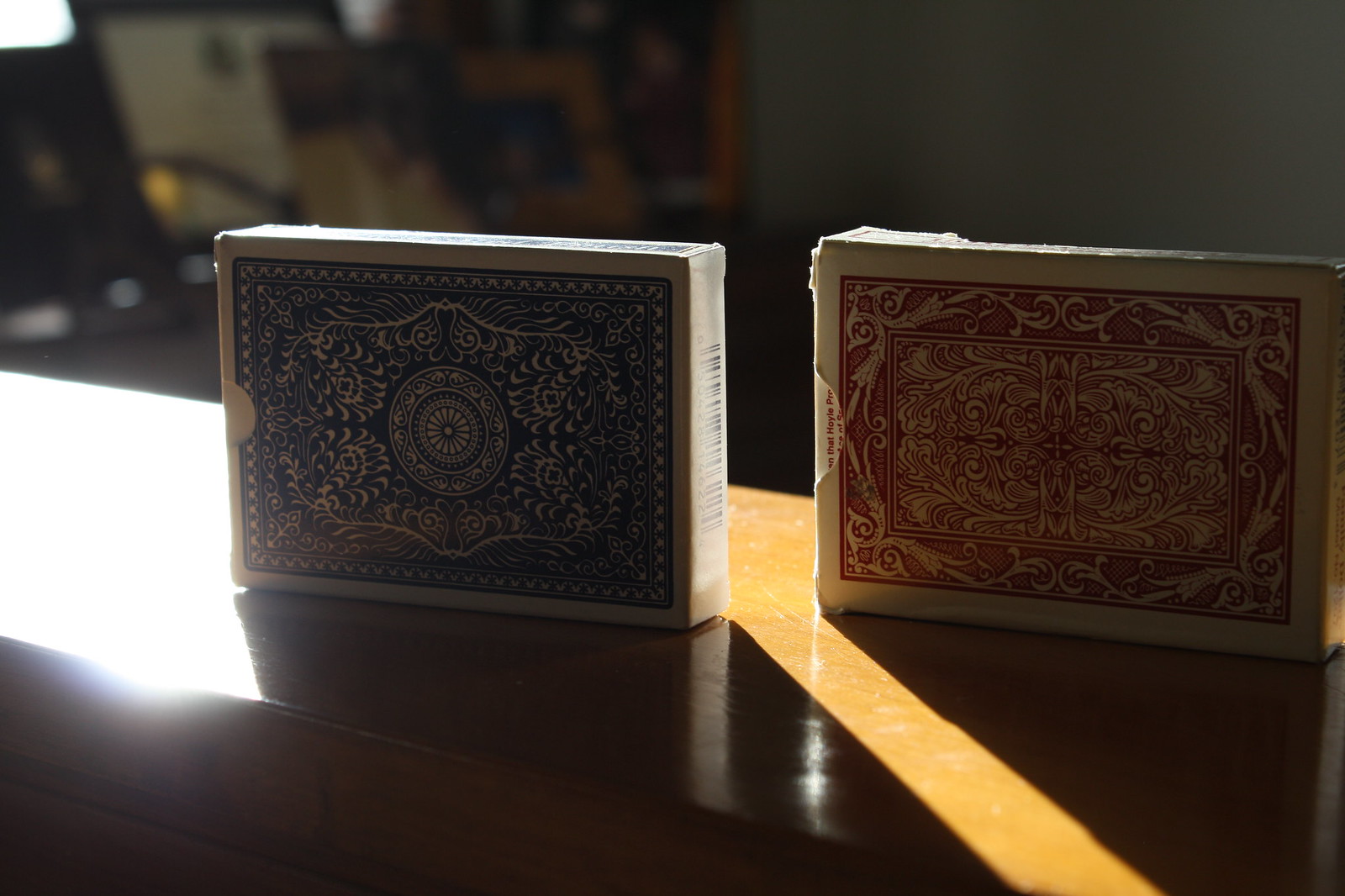The rectangular photograph showcases a light tan-colored wooden mantelpiece. On the mantel sit two decks of cards, still in their packaging, placed vertically. The deck on the left features a bold blue design with a white border. The center of this design has a psychedelic look, with round blue circles and intricate white curves emanating outward. The deck on the right boasts a red design with two vertical red elements that resemble horns, separated by a circle in the middle. Intricate white flames encircle this design in an oval pattern.

Sunlight streams through a window on the left side of the room, casting a distinct shadow on the mantel. This sunlight highlights the space between the two decks of cards, which are separated by about an inch and a half. In the background, to the left of the window, a desk adorned with photographs can be glimpsed, adding depth to the scene. The shadow from the window creates a striking contrast on the wooden mantel, enhancing the vibrant colors of the card decks.